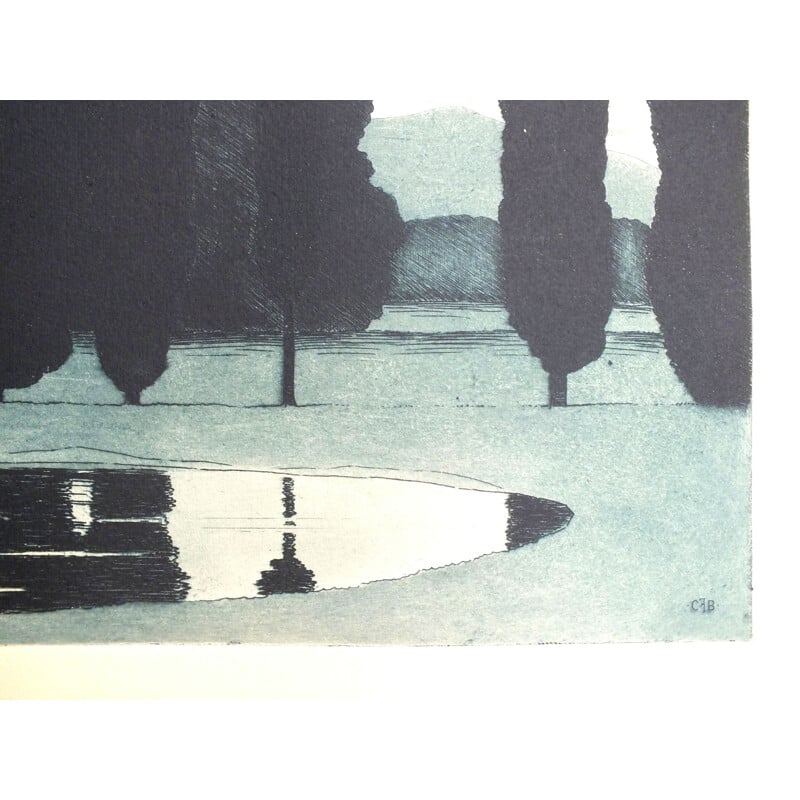This is an image of a hand-drawn sketch, capturing a tranquil, natural landscape primarily in blacks and whites, with hints of gray. The scene features a calm, small lake or pond prominently in the foreground, with intricate reflections of the surrounding environment delicately depicted on its surface. Encircling the pond is an area that resembles grasslands. A row of slender trees, resembling Italian cypress, stands silhouetted against the lighter sky, their narrow trunks and branches reaching skyward. In the background, several hills unfold in layers, the ones nearer to the foreground shaded darker and more scribbled, while those further away blend into the lighter tones of the sky. Additional groves of trees can be seen further behind the main row, adding depth to the landscape. Intriguingly, the entire scene appears to have a slight greenish tint, perhaps a characteristic of the medium used or a scanning artifact. The image is signed in the bottom right corner, decipherable as 'CB'.